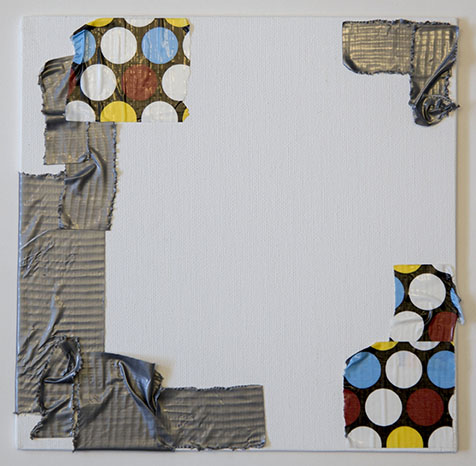The artwork, which appears to be a white canvas or wooden square, features an intricate composition of various duct tapes arranged in a dynamic and textured manner. Dominating the bottom left and top right corners, strips of gray or silver duct tape stretch diagonally across the canvas, with many ridges and air bubbles giving it a rugged texture. Adding a vibrant contrast, pieces of a black duct tape speckled with vivid white, blue, red, and yellow dots adorn the top left corner and reappear in the bottom right, with another smaller piece of the same dotted tape situated directly above. The intersection of these tapes creates a visually engaging collage-like effect while revealing the underlying white surface in untouched areas. The image itself exudes an abstract, multimedia aesthetic, with the vibrant polka dots and the crinkled gray tape creating a striking contrast against the stark white background.